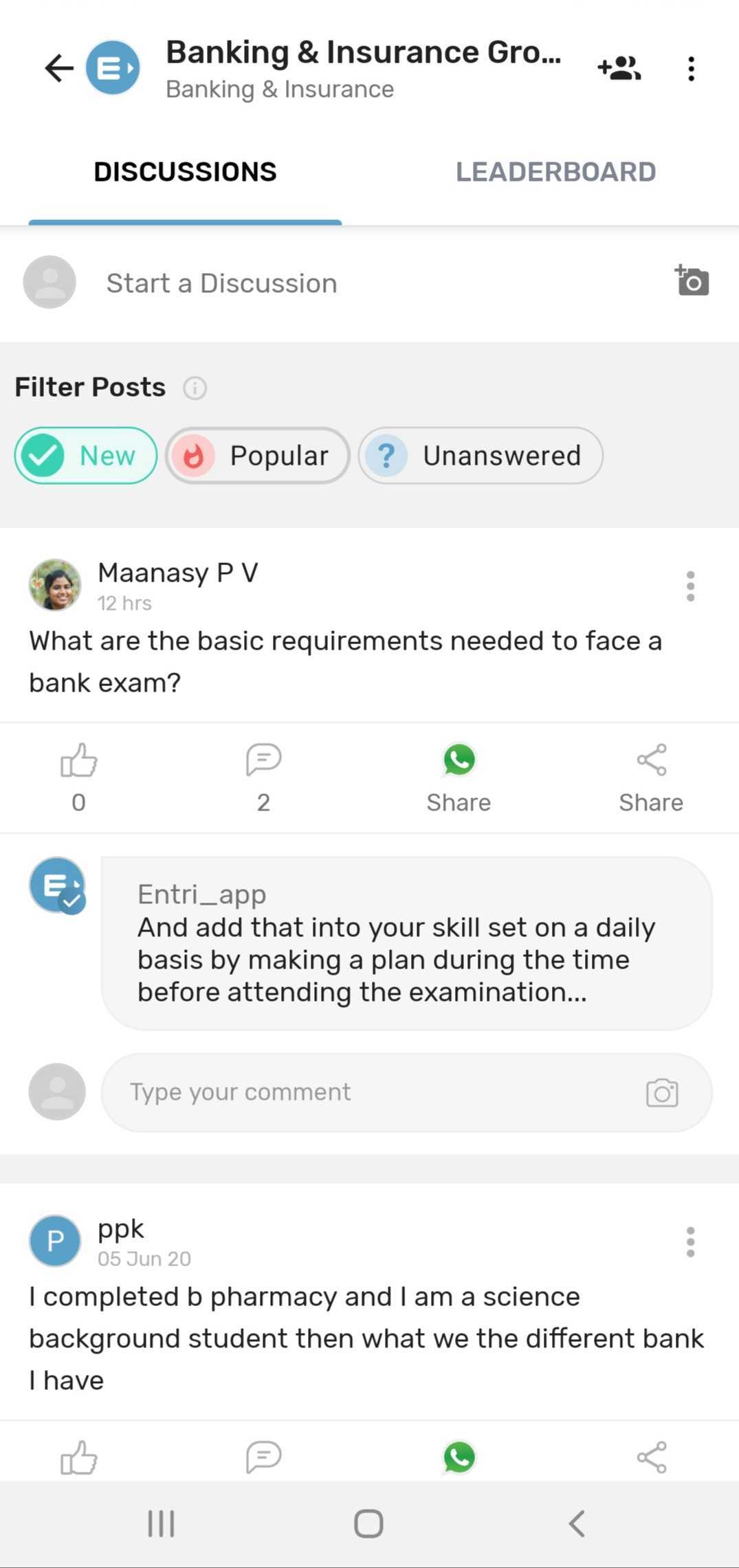This is a screenshot of an app or blog interface, primarily against a white background with some scattered gray boxes. The image is portrait in orientation, significantly taller than it is wide. At the top, a thin gray line demarcates the header from the rest of the page. The header begins with a left-pointing arrow on the top left, followed by a blue circle containing a white capital "E" with a right-pointing arrow next to it. Adjacent to this, the text "Banking and Insurance Group" is displayed, with "banking insurance" written in smaller gray font underneath. There is an icon with two people next to it, indicating an option to add people, followed by a vertical three-dot menu.

Below the header are two scroll options labeled "Discussions" and "Leaderboard." The "Discussions" tab is prominently highlighted in black with a blue underline, indicating it is the active section. The content area begins with an icon of a person and the prompt "Start Discussion." A gray box labeled "Filter posts" allows users to select "New," "Popular," or "Unanswered" posts.

The first visible comment is by a user named Manisapv, asking, "What are the basic requirements needed to face the bank exam?" A subsequent response advises, "Add into your skill set on a daily basis by making a plan during the time before attending the examination." Another comment by a user named PPK mentions something related to pharmacy.